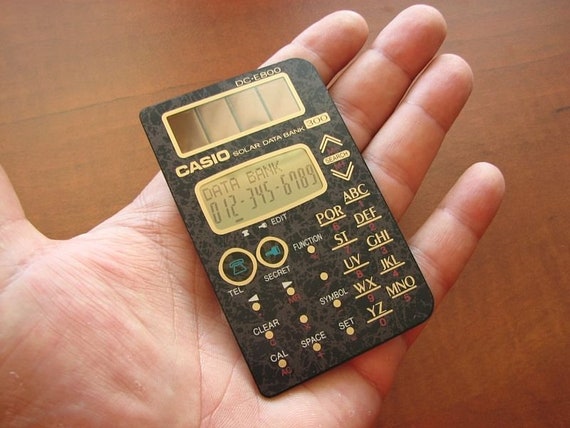The detailed photograph showcases a realistic image, captured by a photographer, of a Casio Solar Data Bank calculator nestled in the open palm of a person's left hand, slightly diagonal. The Casio device, model DC-E800, features a striking red-black marble design with gold-bordered buttons and solar panel. The calculator's screen displays "Data Bank 012-345-6789," and the buttons are adorned with both letters of the alphabet and various functions, including Telephone, Secret, Function, Clear, Calculation, Space, and Set. The remaining buttons are labeled with combinations of letters and numbers such as ABC, DEF, GHI, JKL, MNO, PQRS, TUV, and WXYZ. The photographic background reveals a rich, dark brown wooden table that complements the device's design. A glimpse of intricate details, like the small screen and the clear labeling of the multifunctional buttons, adds to the nostalgic allure of this vintage piece of technology, resembling both a calculator and a possible phone prototype.